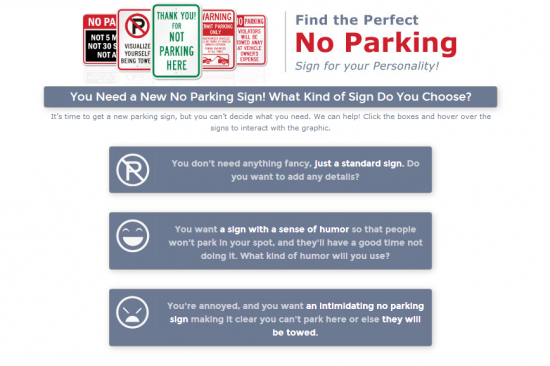**Descriptive Caption:**

The image showcases a series of various parking signs layered on top of each other, starting from the top of the page. From left to right, the first sign is partially visible with a red top section and white font, displaying "No PA," followed by a black section reading "not five," both partially obscured. The next sign prominently features a black "P" with a red slash through it, encircled in red, and a red border. Below the symbol, in black text, the phrase "Visualize yourself being towed" is partly cut off by an overlapping sign.

At the center, a green-bordered sign with a white background stands out, stating "THANK YOU FOR NOT PARKING HERE," with "Not Parking Here" emphasized in larger font. Below it, a sign with "WARNING" in red text and a visual of a car being towed at the bottom is partially visible.

Further down, another small sign reads "No Parking" in white with a red font and border. To the right, a vertical gray line divides the section, above which in gray text reads "Find the Perfect." Following this, "NO PARKING" is displayed boldly in red font. Below in small gray text, "Sign for your personality!" encourages engagement.

Beneath this, a gray rectangular area with white bold text reads, "You need a new no parking sign." Further down, in smaller gray text, the message states: "It's time to get a new parking sign, but you can't decide what you need. We can help. Click the boxes and hover over the signs to interact with the graphic."

Centralized on the page are three horizontally aligned gray rectangles separated by white spaces. The first features a white "P" with a slash through it, captioned with "You don’t need anything fancy, just a standard sign," bolded for emphasis, followed by "Do you want to add any details?"

The second sign shows a smiling face with wide, white teeth and is accompanied by the text, "You want a sign with a sense of humor so that people won't park in your spot and they'll have a good time not doing it. What kind of humor will you use?"

Lastly, an angry smiley face appears next to the statement, "You're annoyed, and you want," followed by a bolded, "an intimidating no parking sign." The final part, not bolded, reads "making it clear you can't park here or else," with the concluding phrase, "they will be towed" emphasized in bold.